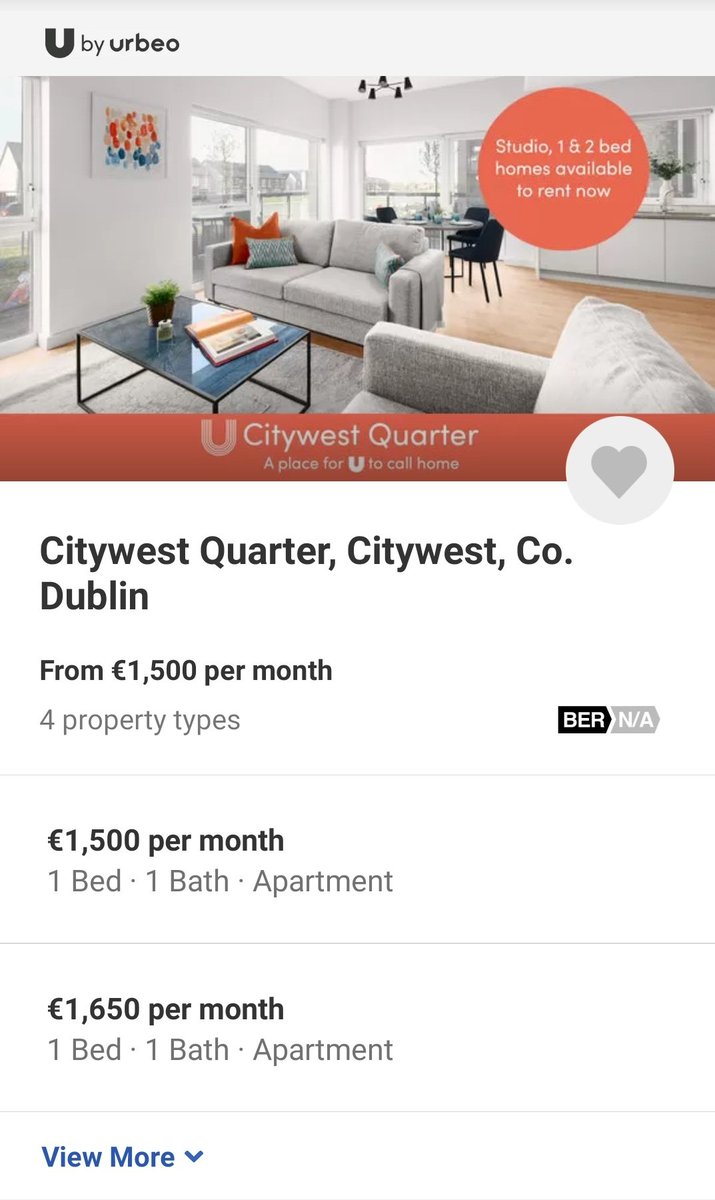The image features a website layout primarily focused on rental properties. At the very top, a gray navigation bar spans the width of the page, with the website name "Urbao" prominently displayed in black lettering on the left side. Below this bar, the main content begins with a photograph of a studio apartment. The apartment is tastefully furnished, showcasing two gray couches facing a coffee table. In the background, there's a dining table accompanied by black chairs.

In the top right corner of the apartment image, a red circular badge with white text announces, "Studio, One, and Two Bed Homes Available to Rent Now." Below the apartment image, a striking red bar stretches across the page, featuring the white-lettered text, "City West Quarter: A Place for You to Call Home." Adjacent to this tagline is a gray circle containing a gray heart icon.

Further down, the page transitions to a white background where additional details about the City West Quarter properties are provided. The text reads: "City West Quarter, City West, Co. Dublin from €1,500 per month for property types," followed by "BER NA." Beneath this, specific pricing information is listed: "€1,500 per month for a one bed, one bath apartment" and "€1,650 per month for a one bed, one bath apartment."

At the bottom of the content, blue lettering invites users to interact with a drop-down menu labeled "View More." This feature allows users to explore different properties that fit their budget and desired location.